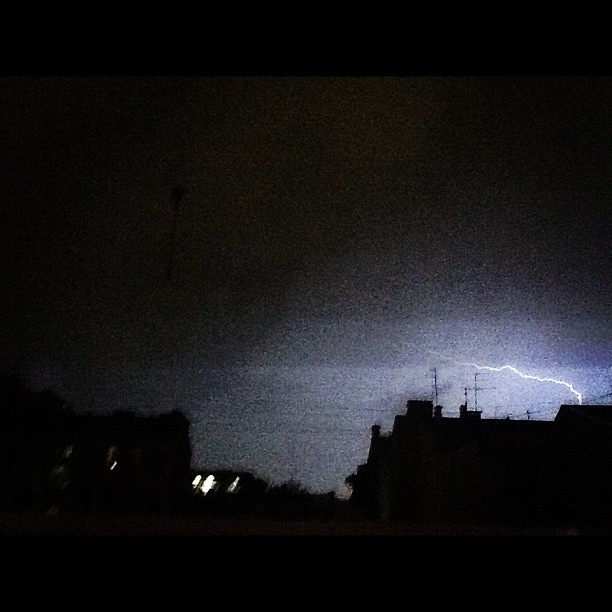The image captures a nighttime scene of a city struck by lightning, enveloped in a pitch-black sky. The primary feature is a single, vivid bolt of lightning striking a building towards the center-right of the image, momentarily illuminating the dark surroundings. Despite the overall blurriness, the silhouette of various square buildings and towers topped with antennas and aerials are visible. Small lights dot the distant landscape, contributing a faint glow. Electrical wires and poles are discernible in the illuminated parts of the sky, accentuating the dramatic, electrifying effect of the lightning against the otherwise impenetrable darkness.